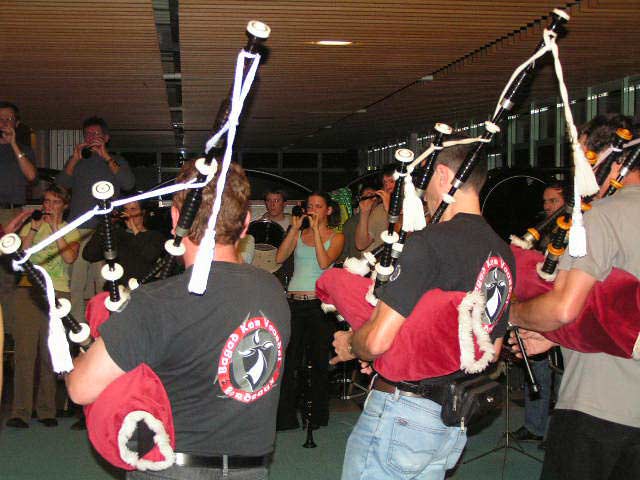Inside a dimly lit venue with a low ceiling, possibly a bar or basement, a crowd has gathered to watch a musical performance. In the foreground, two men are seen from behind, wearing black shirts with a red circular logo, playing Scottish bagpipes. The bagpipes feature red bags with white fluffy outlines, reminiscent of Santa hats, and black pipes adorned with white tassels. These men stand with their backs to the camera, facing an appreciative audience, many of whom are taking photos. The audience, positioned opposite the performers, includes musicians playing various instruments such as flutes and a drum set visible in the background. The room has a cement or tile floor, and the group appears to be arranged in a circle, creating an intimate atmosphere for this lively indoor gathering.